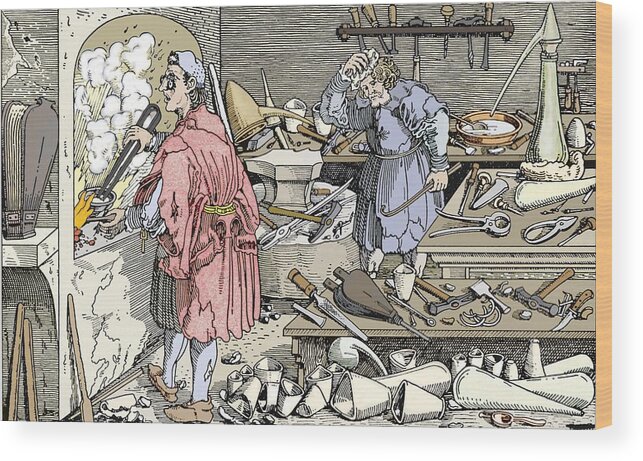This vintage-style illustration, reminiscent of an old-school newspaper cartoon, depicts a chaotic and cluttered workshop or home setting. On the left, a woman dressed in a pink robe and white hat is tending to a wall stove, stirring something over an open flame, with smoke billowing around her. She appears flustered and is wearing black protective glasses. To the right, a man with curly hair and a beard is icing his head with a white bag, wearing a blue long dress and white tights. He holds a crowbar in one hand and is possibly hurt or waiting for the woman to finish. Surrounding them are dark brown tables overflowing with various tools—some that blow smoke, others that chisel, and pliers—adding to the overall sense of disorder in the scene. The detailed tools include items such as wrenches, drills, and fire starters, accentuating the cluttered and chaotic atmosphere.